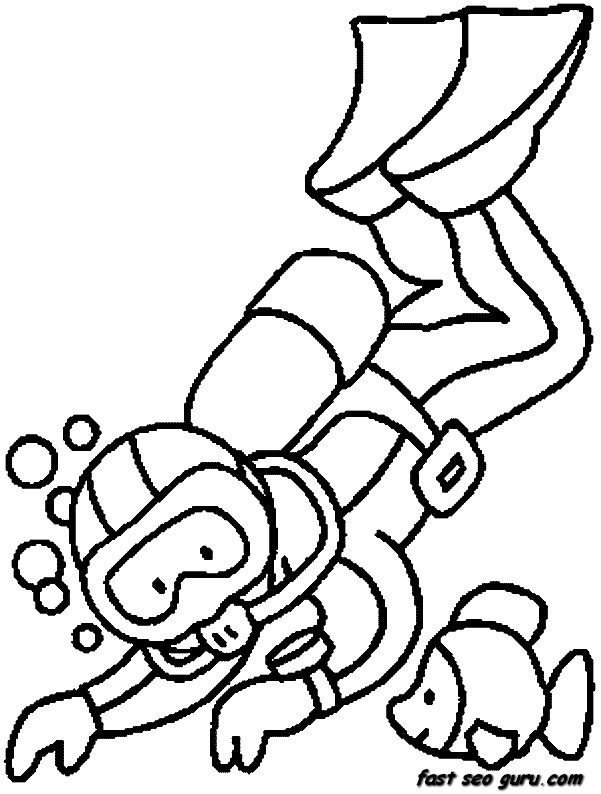The image is a detailed cartoon sketch from a coloring book page, featuring a scuba diver and a fish. The scuba diver is swimming head-first downward towards the lower left corner, with his feet up in the upper right. He wears a full-body wetsuit, flippers on his feet, and a mask with a breathing apparatus connected to an oxygen tank strapped around his lower waist. On his left wrist, there is a watch-like device. Six black-outlined bubbles rise from his mask as he stretches his arms out. The fish, located to the right of the scuba diver's left elbow, has a fin on its top, back, and side, and appears to be smiling with a simplistic dot for an eye. Below the fish, in lowercase black text, is the website "fastseoguru.com." The entire image is rendered in thick lines, making it clear and easy to color.